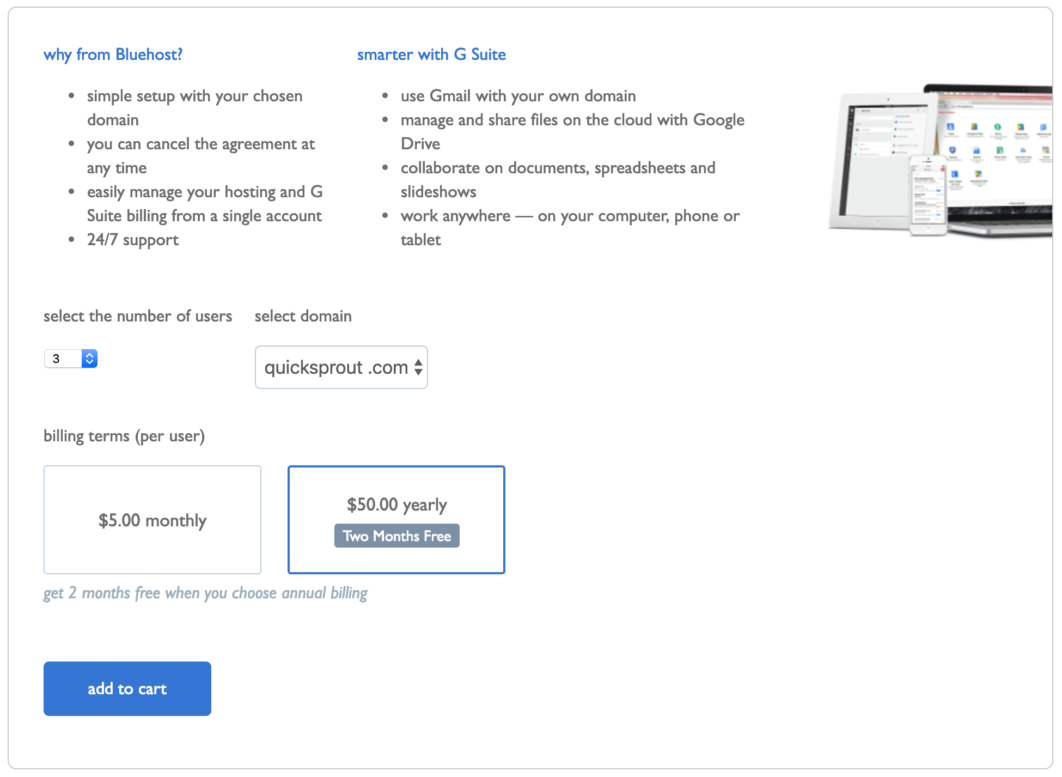The image depicts a detailed promotional infographic from Bluehost, showcasing their integration with G Suite. The outer edge of the image is bordered by a thin, fine line, enclosing a predominantly white background.

At the top, prominently written in blue text, is the headline "Why Bluehost," with 'Bluehost' fully capitalized as one word. Below this heading, a series of bullet points emphasize the key benefits of their service:
- Simple setup with your chosen domain
- Cancel this agreement at any time
- Easily manage your hosting and G Suite billing from a single account
- 24/7 support

Further down, another section in blue font reads "Smarter with G Suite." This section is also supplemented by bullet points detailing the advantages:
- Use Gmail with your own domain
- Manage and share files in the cloud with Google Drive
- Collaborate on documents, spreadsheets, and slideshows
- Work anywhere on your computer, phone, or tablet

Accompanying this text, the infographic features visuals of a computer, tablet, and phone arranged next to each other, illustrating the multi-device compatibility.

Below these visuals, the image provides options for the user to select the number of users and the domain via dropdown menus, which default to three. Following this, a smaller section notes "QuickSprout.com," and outlines the billing terms:
- $5 monthly per user
- $50 yearly per user (normally $60), offering two months free for annual billing

The annual billing option is highlighted with a blue square, and a statement confirms the two months free benefit when choosing annual billing. Finally, the call-to-action button "Add to Cart" is displayed in blue at the bottom of the image.